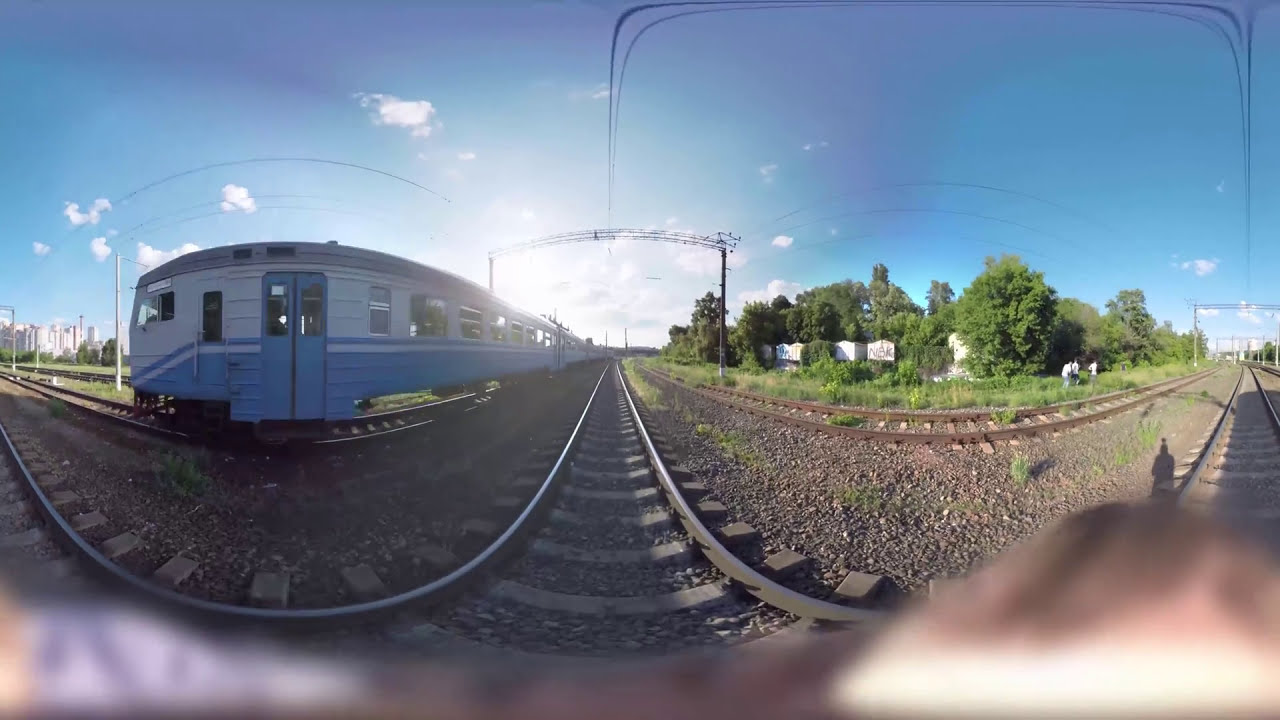The image depicts a distorted, third-vision train scene, likely captured with a 360-degree, stereoscopic, or ultra-wide lens, which lends a conical curvature to the railroad tracks. The bottom middle of the photo features these tracks, curving due to the lens distortion, and extending through varied landscapes. On the right middle half, there is a country scene with a grove of green trees, overhanging electric train wires, and possibly some shops nestled among the trees. To the left, the scene transitions into an urban landscape, with a blue and white train prominently visible on the distorted tracks. The train, appearing warped and making an illusory left-hand turn, accentuates the image's surreal quality. The train's doors and bottom half are blue, while the top half is white. Above, a very blue sky, dotted with scattered small white clouds, stretches with the sun almost dead center, illuminating the bottom third of this vivid sky. The photo also captures the shadow of the photographer in the far right lower part, adding a unique dimension to the image. The lower portion of the image is blurred, possibly due to the camera or the photographer's hand. The sky features hints of purple, particularly around the horizon, emphasizing the time—either sunrise or sunset—through the warm glow spreading across the scene.